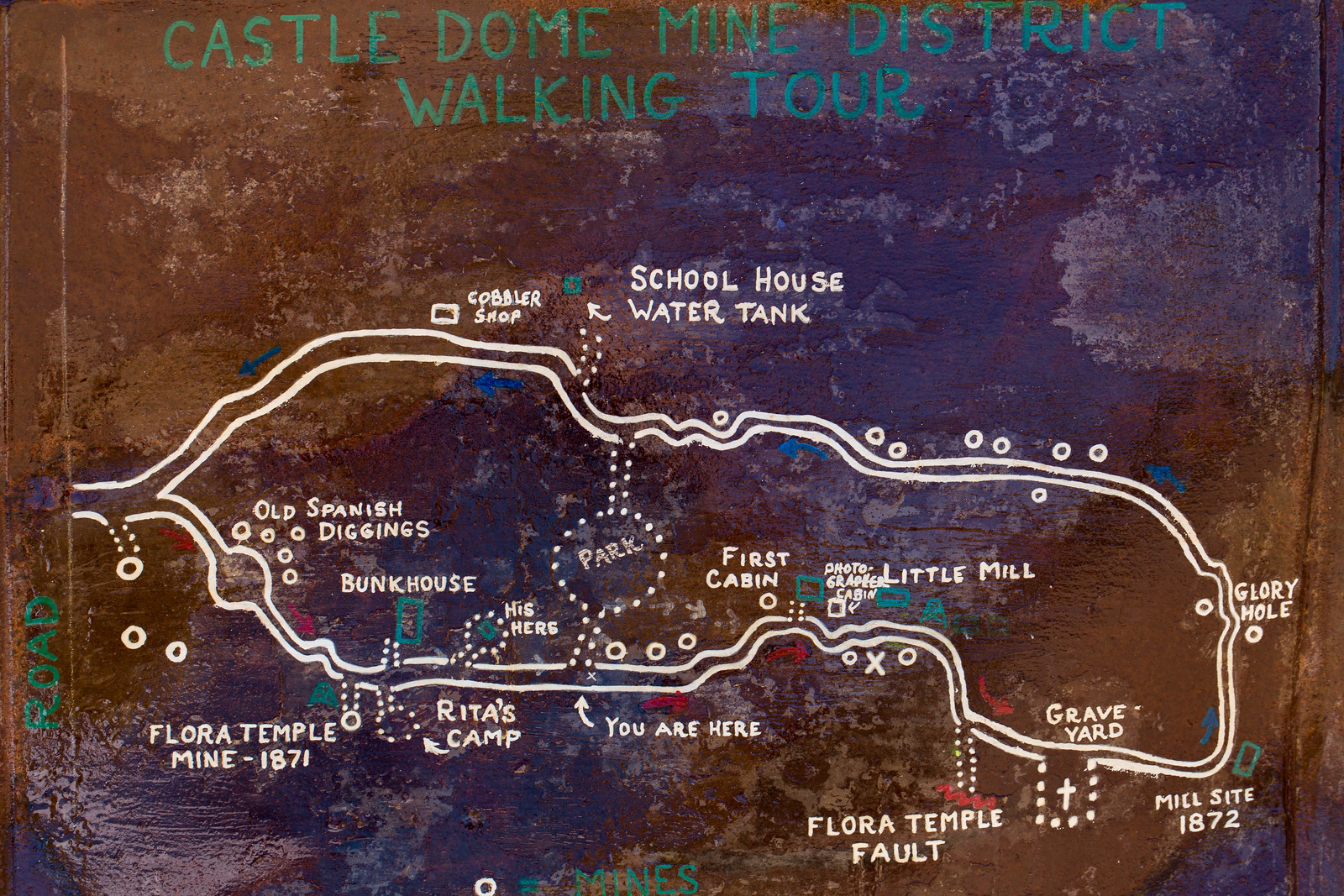The photograph captures a hand-drawn, detailed map mounted on a cement wall, titled "Castle Dome Mine District Walking Tour" in green text at the top. The map itself, displayed on a brown background, features a circular path outlined in white. This path guides visitors through various historical and significant locations such as the Cobbler Shop, Schoolhouse Water Tank, Glory Hole, Mill Site, Graveyard, Flora Temple Fault, Little Mill, First Cabin, Rita's Camp, Bunkhouse, Flora Temple Mine, and Old Spanish Diggings. A notable feature includes a marker indicating "You Are Here." In the middle of the circular path is a dotted area designating parking space. The map combines white paint for the trail and labels, with occasional green and red boxes highlighting specific points of interest, encapsulating a rustic and informative walking tour experience of the Castle Dome Mine District.